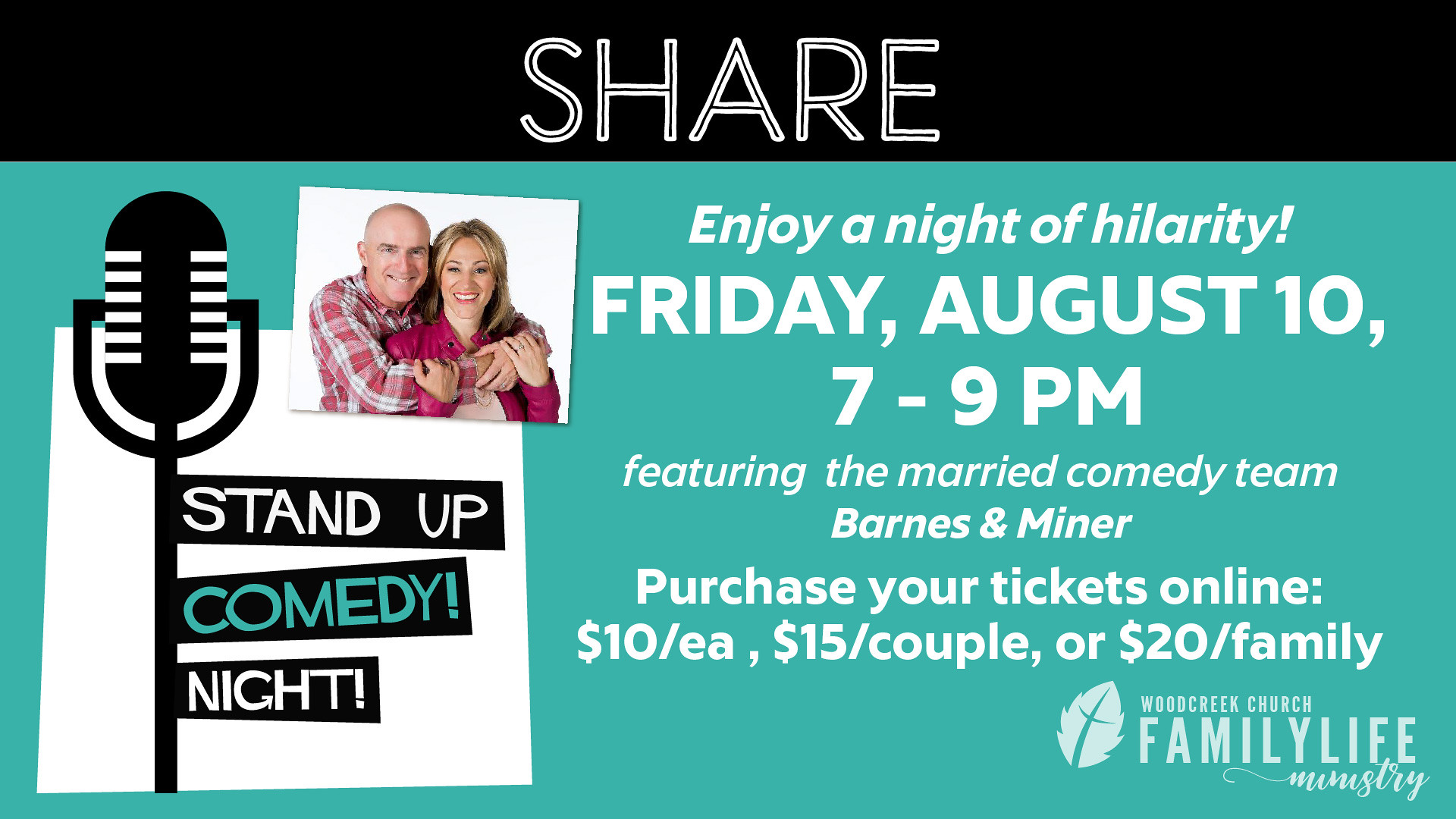This color photograph, combined with graphic design and typography, showcases an advertisement in landscape orientation, promoting a comedy event. Central to the image is a photograph of a smiling man and woman; the man, bald and dressed in a white and red checkered shirt, is embracing the woman, who has shoulder-length hair and wears a pink shirt. They both gaze joyfully at the camera, highlighting a sense of warmth and connection. Above them, a black horizontal strip features the word "Share" outlined in white. 

To the left of the photo, a black line-art microphone on a stand introduces the event with text on a black background reading "Stand Up Comedy Night!" To the right, in white text, it reads, "Enjoy a night of hilarity! Friday, August 10th, 7-9pm. Featuring the married comedy team Barnes & Minor." Below this, ticket pricing is detailed: "$10 each, $15 a couple, or $20 a family. Purchase your tickets online."

The bottom right features the logo of Woodcreek Family Life Ministry with a feather symbol crossed by a line. This image effectively combines photographic representationalism and graphic design to create an engaging and informative advertisement for the comedy night.